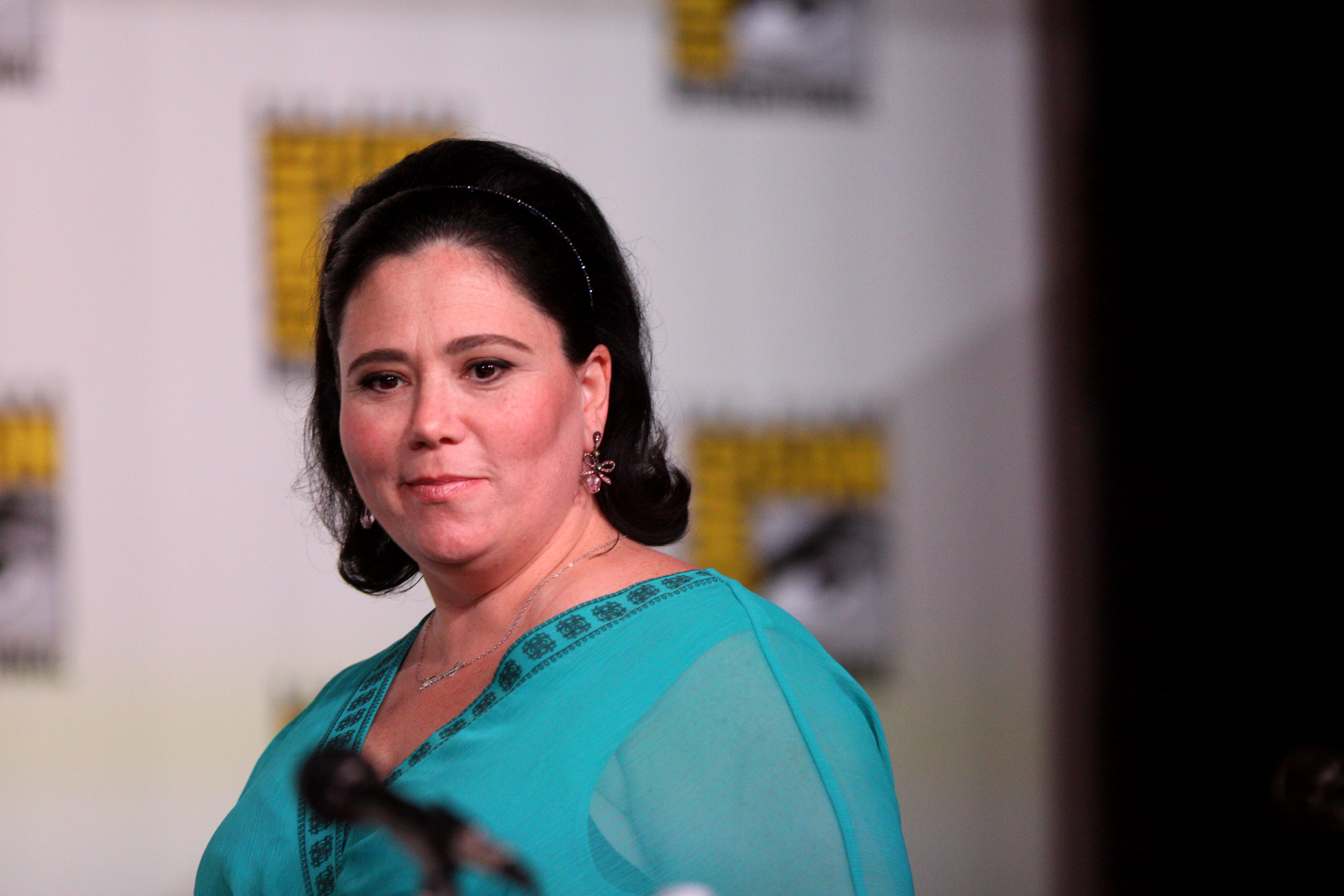This photo captures actress Alex Borstein at Comic-Con, standing against a white backdrop emblazoned with the Comic-Con logo, which fades into darkness on the right side, suggesting an offstage area. Alex is dressed in a bright turquoise dress with sheer green sleeves, complemented by black accents along the neckline, which is shaped in a V-formation. She accessorizes with a thin silver necklace and a pair of dangling earrings that resemble bows with gems beneath them. Her dark brown hair, adorned with a simple hairband, falls to her shoulders, pairing seamlessly with her equally dark brown eyes. Although her gaze is directed slightly downward toward another camera, giving her a candid and unposed appearance, the composition highlights her as the focal point, standing in sync with the event’s energetic atmosphere. A blurry microphone is positioned in front of her, hinting at a possible interview or panel discussion at the event. The scene emphasizes her natural beauty with minimal makeup, underscoring a modest yet elegant presence fit for the occasion.